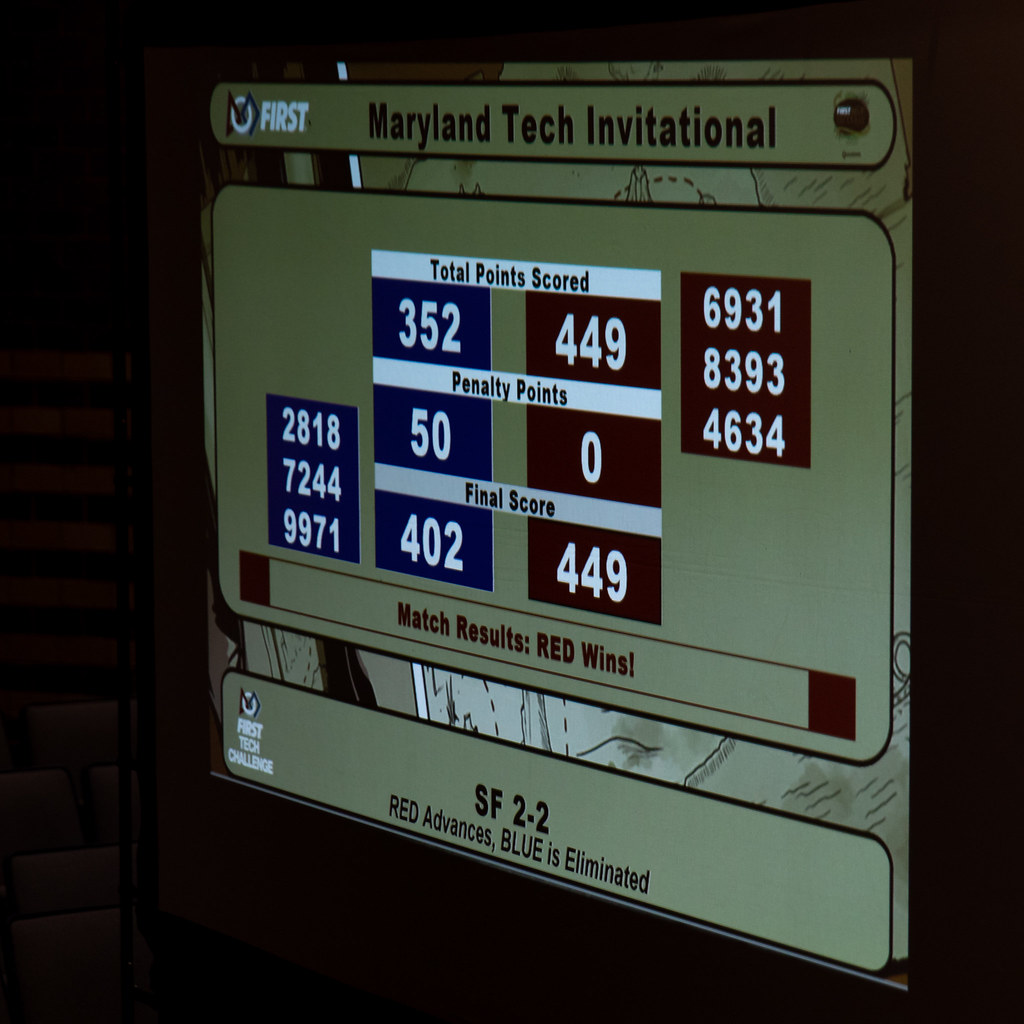The photograph captures a dimly lit indoor setting, predominantly dark with shadowy areas on the periphery, focusing on a brightly illuminated scoreboard in the center. At the top of the scoreboard, it reads "FIRST" in white, accompanied by a logo, followed by "Maryland Tech Invitational" below in black. The scoreboard, primarily light brown or tan with black framing, displays "TOTAL POINTS SCORED" prominently in white. On the left, the blue section shows "352," while the red section on the right lists "449." Underneath, it details "PENALTY POINTS" in black, with the blue box indicating "50" and the red box showing "0." The "FINAL SCORE" section shows "402" in blue on the left and "449" in red on the right. Additionally, beneath the corresponding scores, blue rectangles list the numbers "2818," "7244," and "9971," while red rectangles display "6931," "8393," and "4634." At the bottom, within a red-outlined rectangle, the text "MATCH RESULTS" states "RED WINS" in red, and further down, "SF2-2," "RED ADVANCES," and "BLUE IS ELIMINATED" are inscribed in black. The scoreboard stands out vividly against the dark and somewhat obscure background, making it the focal point of the photograph.